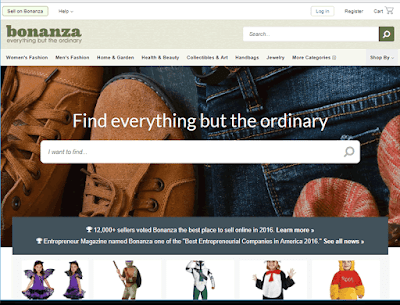This screenshot from a web page features the online store Bonanza. At the top of the page, the title "Bonanza" is displayed in all lowercase letters with a pale green background and dark green font. Below the title, there are eight navigational categories listed horizontally, though the text is too small to be legible. A search bar is also prominently positioned at the top of the page.

The main content below the categories includes a photograph mainly showing a section of denim jeans, highlighted by visible stitching and a belt loop, suggesting a back pocket area. Additionally, a pair of boots is partially seen. At the bottom of the page, there are images of children dressed in various Halloween costumes, including characters like Winnie the Pooh, a fairy, and possibly a penguin. The overall layout and visual elements encapsulate a diverse range of items and themes associated with the Bonanza website.